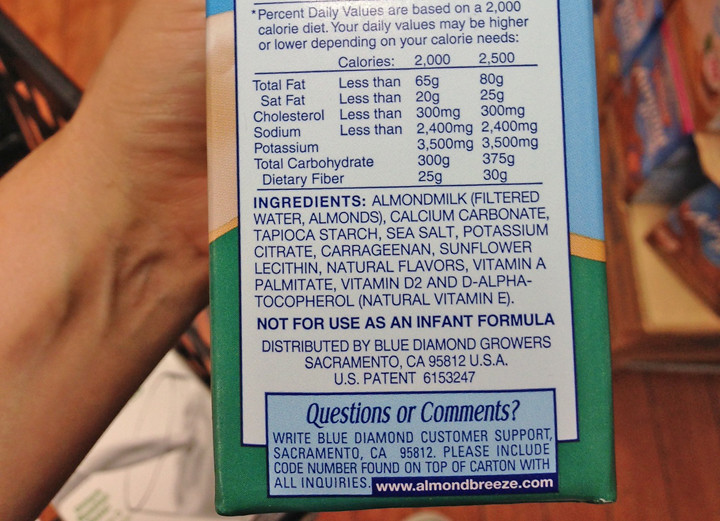The image captures the back of an Almond Breeze brand almond milk container, oriented horizontally. In the foreground, a left hand is visibly holding the container, with the wrist positioned on the left side of the image and the palm facing the viewer. The backdrop reveals various household elements, including a wooden floor and a stack of almond milk containers on the right side.

The nutritional label on the container begins with a note that the percent daily values are based on a 2,000 calorie diet, advising that individual daily values might differ based on personal dietary needs. Listed nutritional information follows, detailing fat, cholesterol, and other vital components. The ingredients section, which includes items such as almond milk, filtered water, almonds, and calcium carbonate, is also visible. One notable detail on the label is a disclaimer stating the product is not for use as an infant formula. Additionally, at the bottom of the label, enclosed in a blue box, there's information for inquiries and comments with the website www.almondbreeze.com provided.